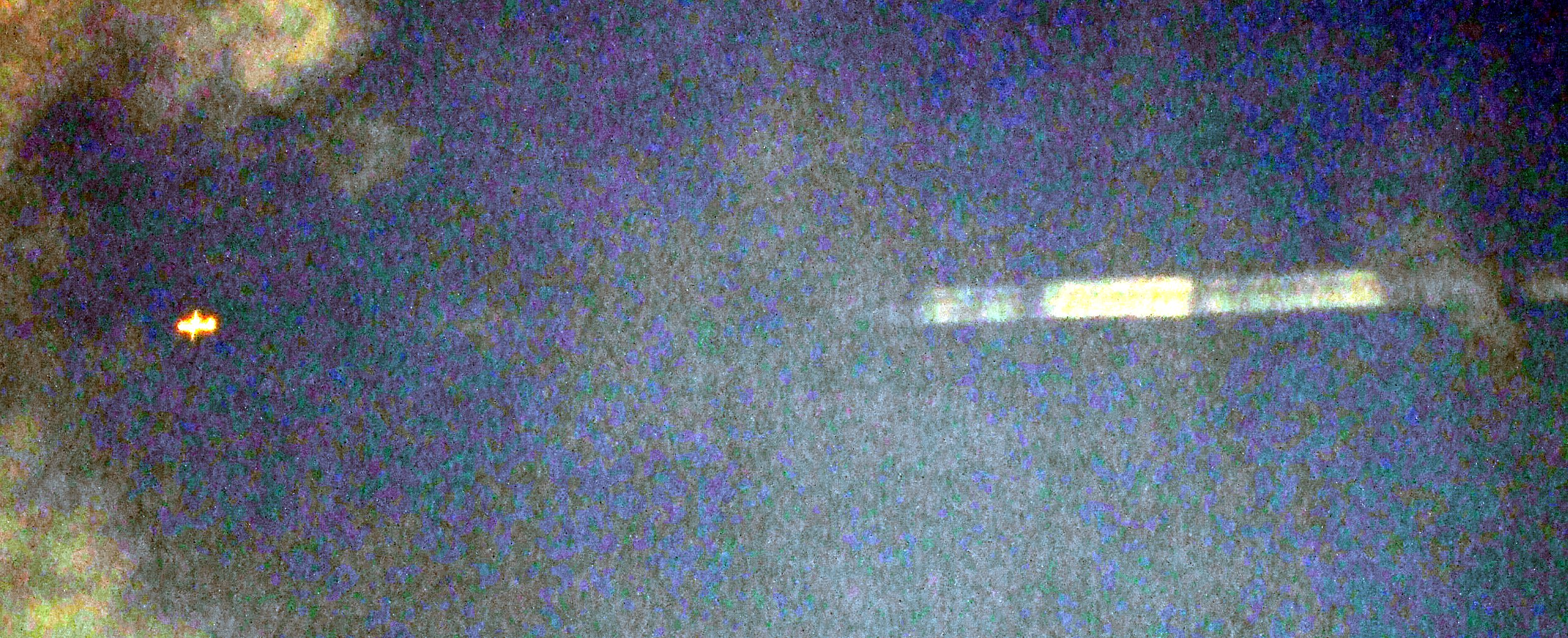The photograph is a highly pixelated, rectangular satellite image primarily in deep blue shades, depicting an aerial view of an ocean. The vast majority of the image is a continuum of blue with intermittent spots of green and gray, transitioning on the left side into more yellow and darker gray hues. Dominating the center-left, there is a glowing, orange-white object that resembles a small plane or possibly a missile, with tiny protrusions that could be wings, though its blurred, radiant appearance obscures finer details. Extending from this object towards the middle right of the image is a hazy white and yellowish line, hinting at a possible path or trail left by the moving object. The right side of the image, horizontally centered, features a series of indistinct, blurry white squares, contributing to the overall pixelated and grainy quality of the photograph. The sky around the object is an ominous blend of purplish-blue, accentuated by sporadic clouds, particularly around the left half of the image where the glowing object is situated.